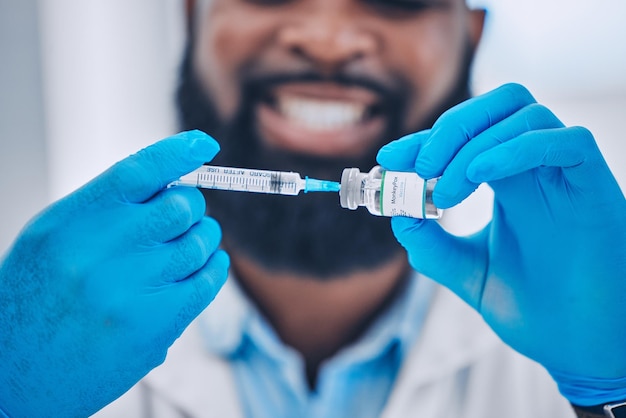In this detailed photograph, a man, presumably a medical professional, is shown drawing liquid from a vial labeled "monkey pox" into a syringe. The man has dark skin, a thick black beard, and a mustache, and he is smiling broadly, showing all of his teeth, although his facial features are somewhat out of focus. He is dressed in a white lab coat over a baby blue dress shirt and is wearing sterile blue latex gloves that hold the vial and syringe prominently in the foreground. The vial has a white label with a green outline, and the syringe features a blue tip and black writing along its side. The meticulous focus on the gloved hands holding the vial and syringe suggests an emphasis on the vaccination process. The image is cropped just below the man's eyes, with a white background that keeps the attention on the detailed action of the hands preparing the monkey pox vaccine.